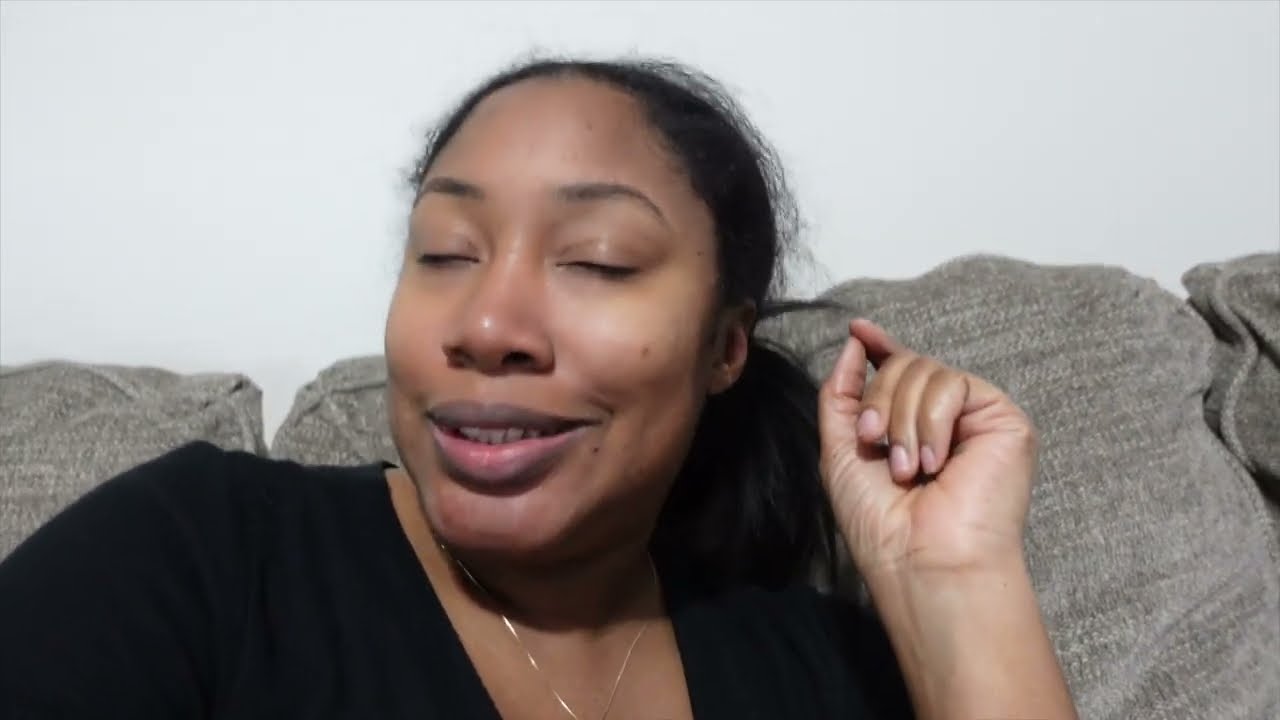In the image, an African-American woman with her eyes closed is sitting on a gray couch with three thick, comfortable-looking cushions behind her. Her black hair is pulled back into a ponytail, and you can see it hanging down towards her shoulders. She is wearing a black v-neck shirt and a very thin necklace, either gold or silver, shaped in a v around her neck. The woman is smiling, showing little dimples in her cheeks, and her left hand is raised near her ear with her thumb and pointer finger pinched together, while her other fingers are curled into a fist, palm facing forward. Behind her is a light gray or whitish wall. The image, potentially a screenshot from a video call, focuses on her engaging expression and posture.